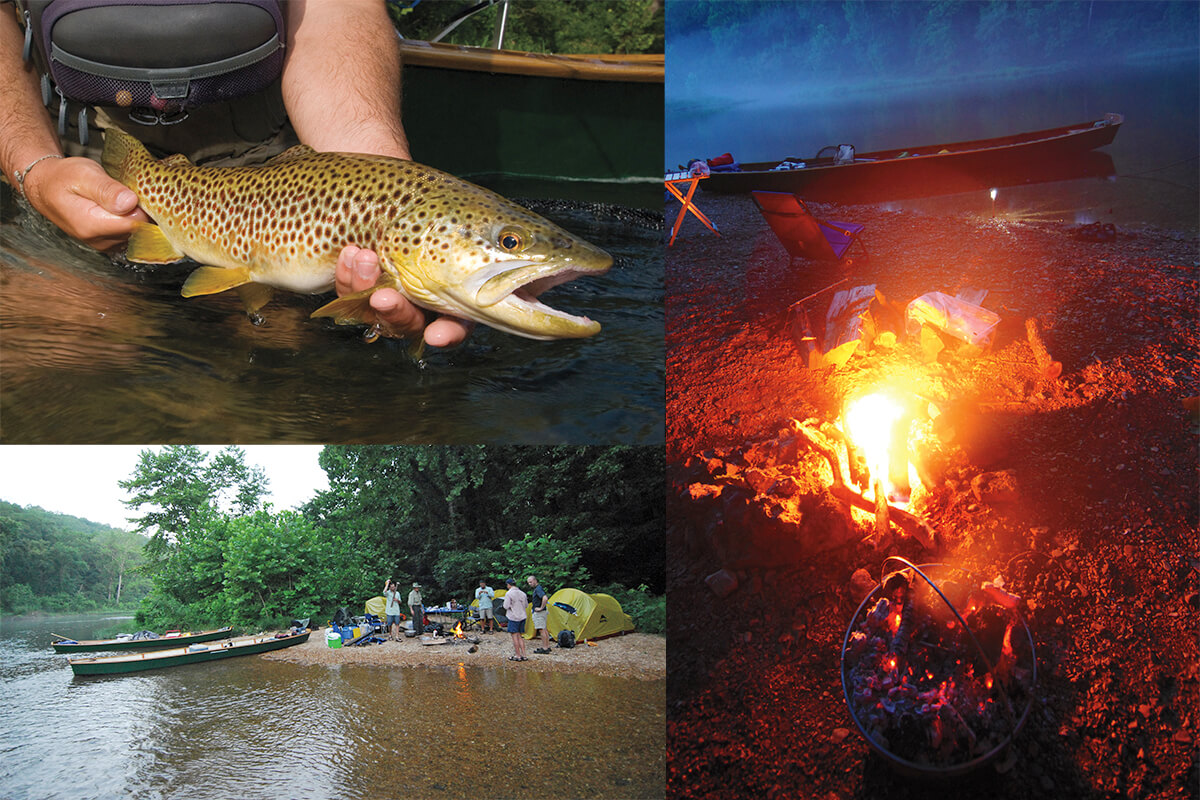The image is composed of three distinct photos, with the right-hand photo taking up half of the overall image and the two photos on the left-hand side taking up the other half, stacked vertically. 

In the top left photo, a Caucasian individual wearing black clothing is holding an olive-colored fish with brown eyes and black spots just above the water. The person's chest area is partly visible, and in the background, there is a brown boat. 

Below, the bottom left photo showcases a lush, green wooded area by the edge of a river or creek. On the sandy beach, five people are busy setting up camp. They have erected several green tents and have some camping gear scattered around, along with two beached long canoes. A vivid orange campfire is ablaze as part of their campsite setup.

The right-hand photograph seems to capture a continuation of this camp scene but taken at night. A glowing bonfire, emitting orangish-red flames, is the focal point. Chairs, including a notable blue one in the foreground, are set up around the fire. In the background, a boat can be spotted by the water's edge, with the darkened river and surrounding forest contributing to the night-time ambiance.